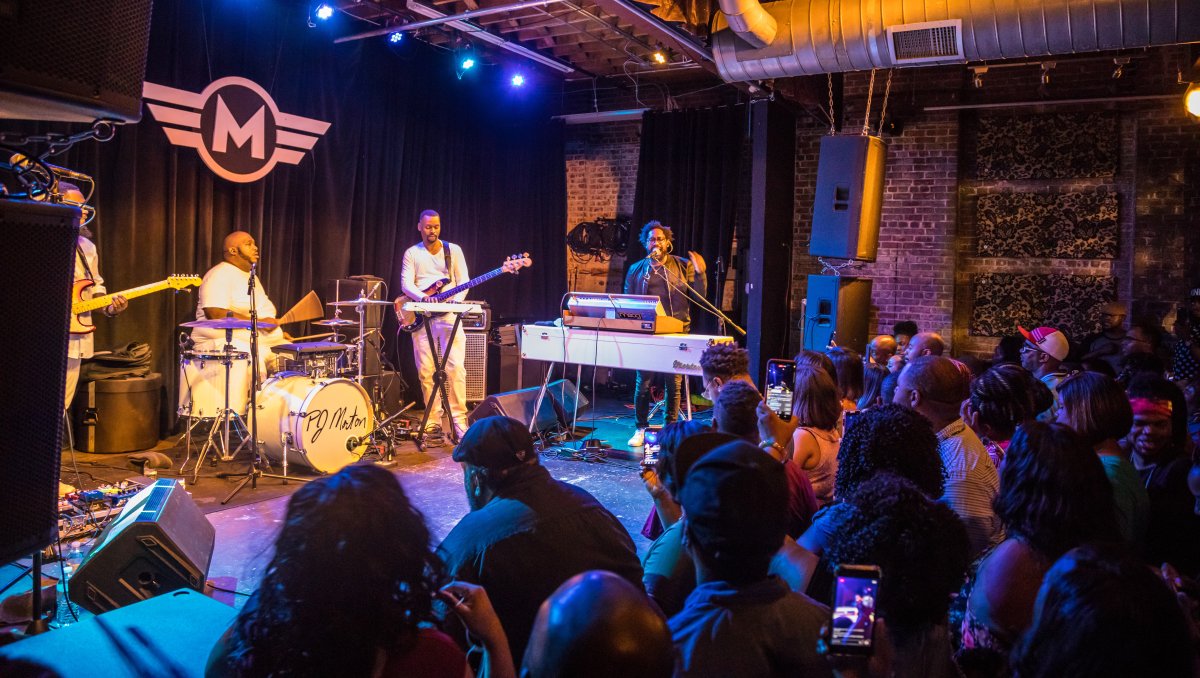In this image, captured in landscape orientation, we see a vibrant live concert set in an indoor venue with exposed brick walls and an unfinished ceiling featuring visible HVAC tubes. The stage, positioned towards the left half of the picture, hosts a diverse band with several musicians. From right to left, there is a keyboardist with a microphone, passionately singing or speaking, followed by a bassist, a drummer seated behind a kit that reads "PJ Minton," and a lead guitarist. Behind the band, black curtains serve as a backdrop, adorned with a distinct logo: a capital 'M' encircled and flanked by three horizontal lines on each side, resembling wings. Various amplifiers and speakers are strategically placed around the stage to enhance the sound.

In the bottom right quadrant, the audience is visible, albeit in shadow, attentively watching the performance. Some people in the crowd are seen capturing the moment with their phones. The photographer's vantage point, slightly elevated above the crowd, offers a comprehensive view of the band and the audience, encapsulating the lively atmosphere of the concert at this intimate club setting.